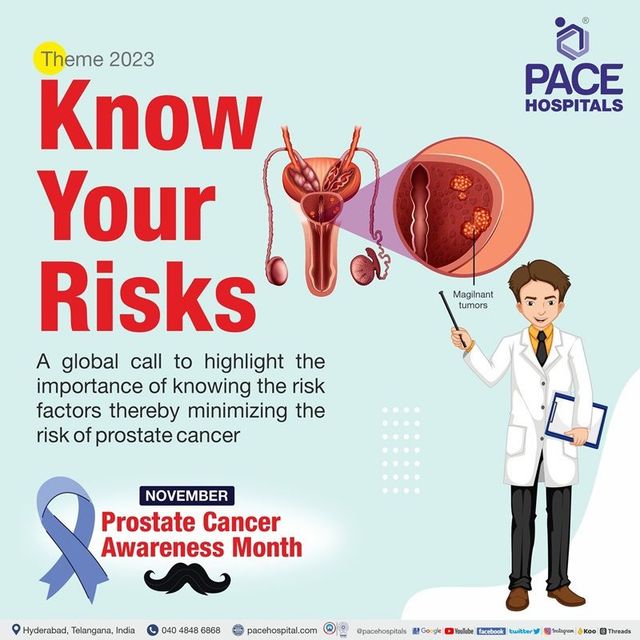This is a detailed, color public service poster on a light blue background, primarily promoting awareness of prostate cancer risks. Dominating the upper left corner is the headline in large red text: "Know Your Risks." Beneath it, in smaller black text, the poster reads: "A Global Call to Highlight the Importance of Knowing the Risk Factors, Thereby Minimizing the Risk of Prostate Cancer." Adjacent to this text is a detailed diagram of the prostate, illustrated in shades of pink, red, peach, and purple, with a circular inset providing further details. Below the diagram stands a cartoon doctor in a white lab coat, holding a clipboard in one hand and pointing to the prostate diagram with a pointer in the other. 

In the lower left section of the poster, a blue ribbon — symbolizing prostate cancer awareness — appears with white text that states "Prostate Cancer Awareness Month." Positioned inside a black background, the word "November" is highlighted in white text, and a black mustache is prominently featured below it, reinforcing the awareness theme often associated with Movember. 

The upper right corner bears the logo of Pace Hospitals in purple, suggesting they are the sponsor. Additionally, small text at the bottom of the poster provides addresses and phone numbers. In the top center, there is also a reference to "Theme 2023" marked by a yellow circle around the letters "TH."